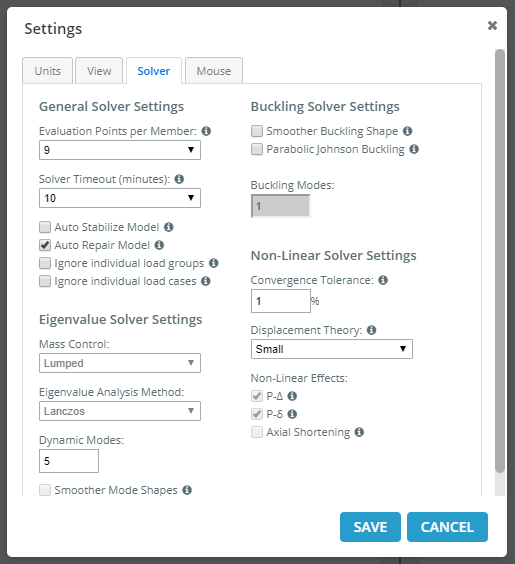The image depicts the settings menu of a software application. The word "Settings" is prominently displayed in black font with a capital "S" in the upper left-hand corner. To the upper right, there is a 'Close' button indicated for exiting the menu.

The menu has four tabs: Units, View, Solver, and Mouse. The currently selected tab is "Solver". Under this tab, there are several options for configuring the solver settings.

1. **General Solver Settings:**
   - **Evaluation Points per Member:** 9
   - **Solver Timeout (minutes):** 10

2. **Checkbox Options:**
   - **Auto Stabilize Model** 
   - **Auto Repair Model** (checked)
   - **Ignore Individual Load Groups**
   - **Ignore Individual Load Cases**

3. **Solve Setting:**
   - **Mass-Control:** Lumped

4. **Analyst Method:**
   - **Lanczos**
   
5. **Dynamic Modes:** 5
6. **Buckling Modes:** 1

The interface is designed to allow users to finely tune solver parameters to match their simulation requirements.